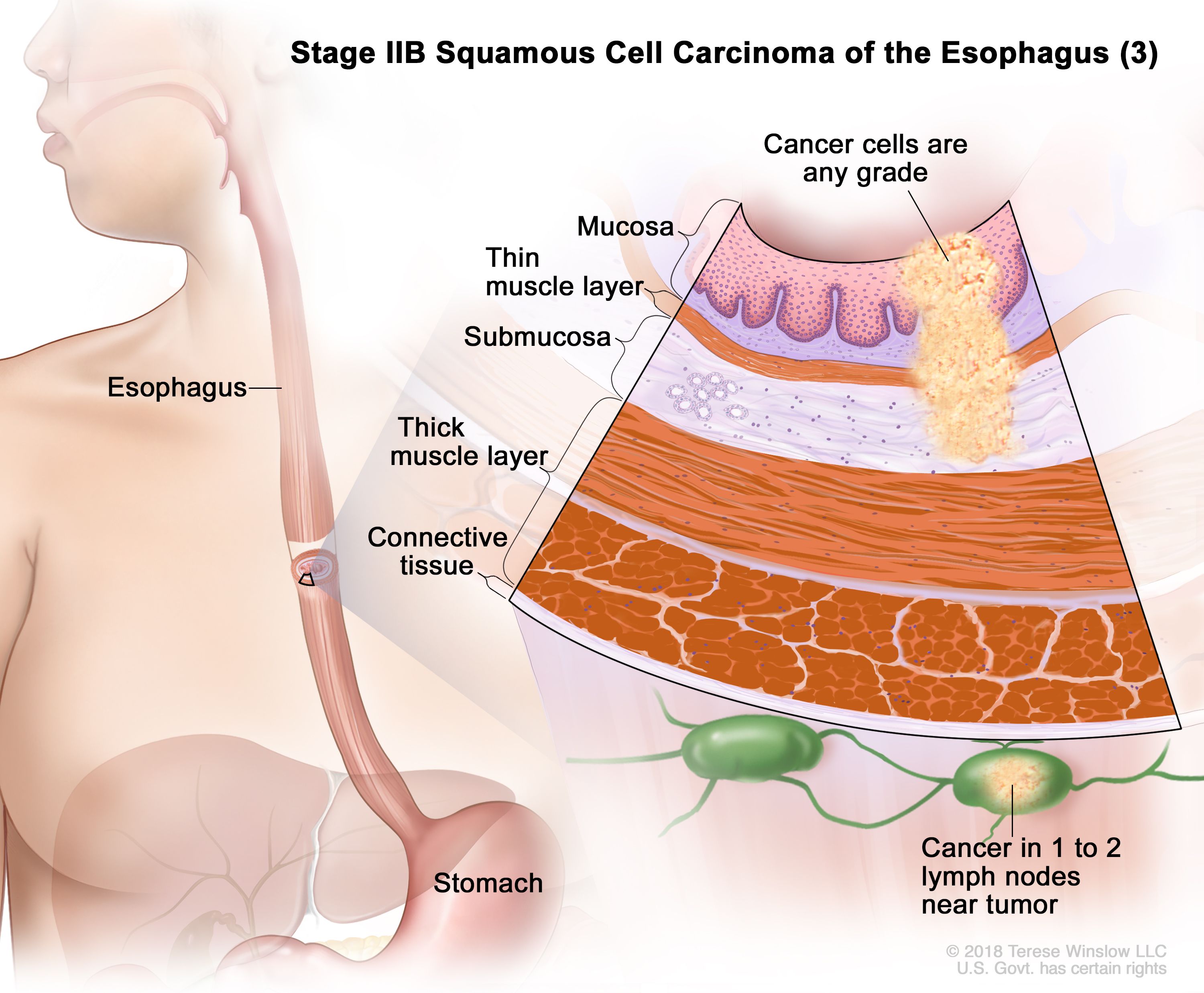The image is a computer-generated medical diagram with a white background that illustrates and labels critical aspects of Stage IIB squamous cell carcinoma of the esophagus. At the top center, the title is written in black text: "Stage IIB Squamous Cell Carcinoma of the Esophagus [3]."

On the left side of the diagram, there is a profile view of a human body, highlighting the esophagus as a red tube extending from the mouth to the stomach. This section shows the anatomical path of the esophagus and its connection to the stomach, providing a contextual overview of the affected region.

To the right of this anatomical illustration is a detailed cross-sectional view of the esophagus at the cellular level. This section is organized into labeled segments illustrating the different tissue layers:

- **Mucosa**: Illustrated as a light pink layer with a jagged bottom edge.
- **Thin Muscle Layer**: A thin red line beneath the mucosa.
- **Submucosa**: A white area populated with small dots below the thin muscle layer.
- **Thick Muscle Layer**: Depicted as a solid red area.
- **Connective Tissue**: A section with red and light pink striping below the thick muscle layer.

At the top of this cellular diagram, a yellow cone shape with yellow dots represents cancer cells of any grade. Additionally, beneath this illustration, green, oval-shaped structures labeled as "cancer in 1 to 2 lymph nodes near the tumor" are depicted, resembling bugs or ticks, symbolizing the spread of cancer to nearby lymph nodes. The overall layout and details provide a comprehensive visualization of the anatomy and pathology associated with esophageal squamous cell carcinoma.